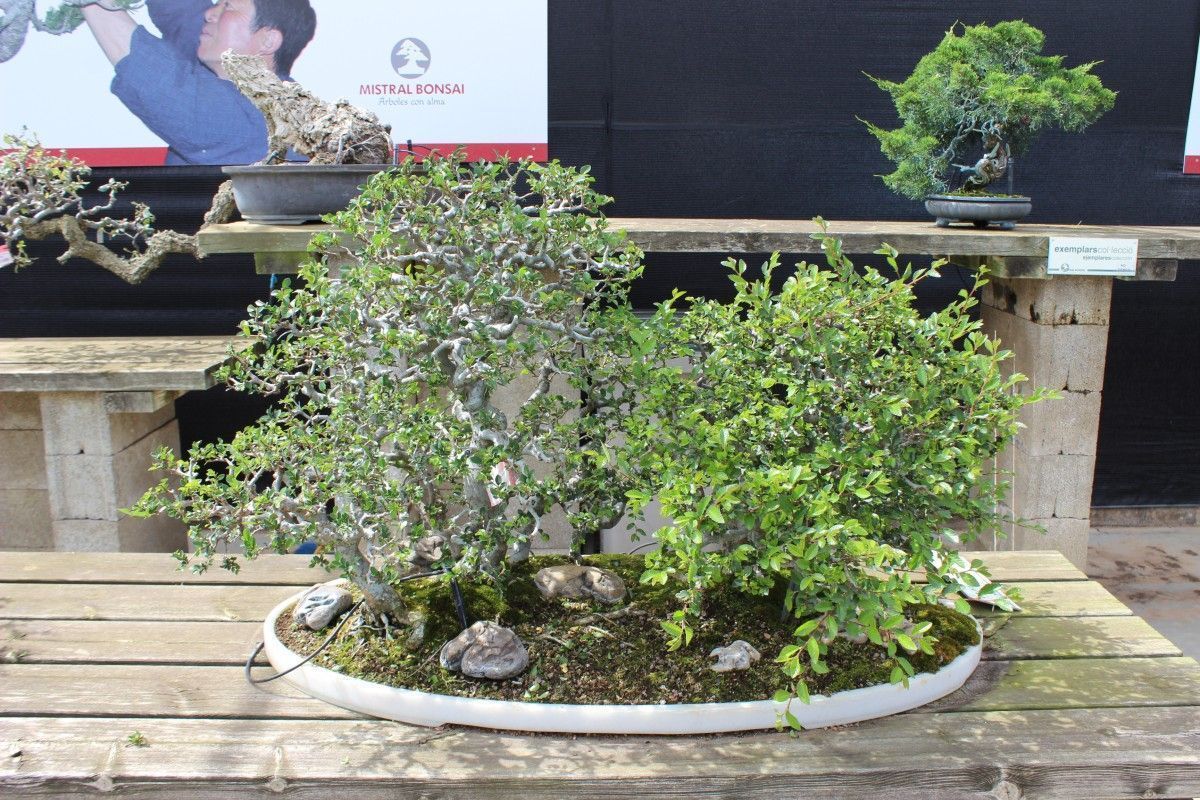This detailed photograph captures an outdoor setting during the day, featuring a couple of bonsai trees. In the foreground, two bonsai trees reside in a shallow, oval-shaped white container filled with soil and miniature rocks. The tree on the left is taller, with green leaves tinged in white, while the one on the right is shorter and denser, flaunting bright green leaves. This container rests on a horizontal brown wooden bench.

In the background, there are two other benches of different heights. The higher bench houses two more bonsai trees in shallow, wide green bowls. The tree on the left has a branch extending across to the edge of the image, while the tree on the right is notable for its bright green leaves. A white and red sign reading "Mistral Bonsai" can be seen, along with some partially readable black lettering, possibly "publica.com".

Overall, the scene is carefully composed to showcase the intricate details of the bonsai trees within their serene outdoor setting.